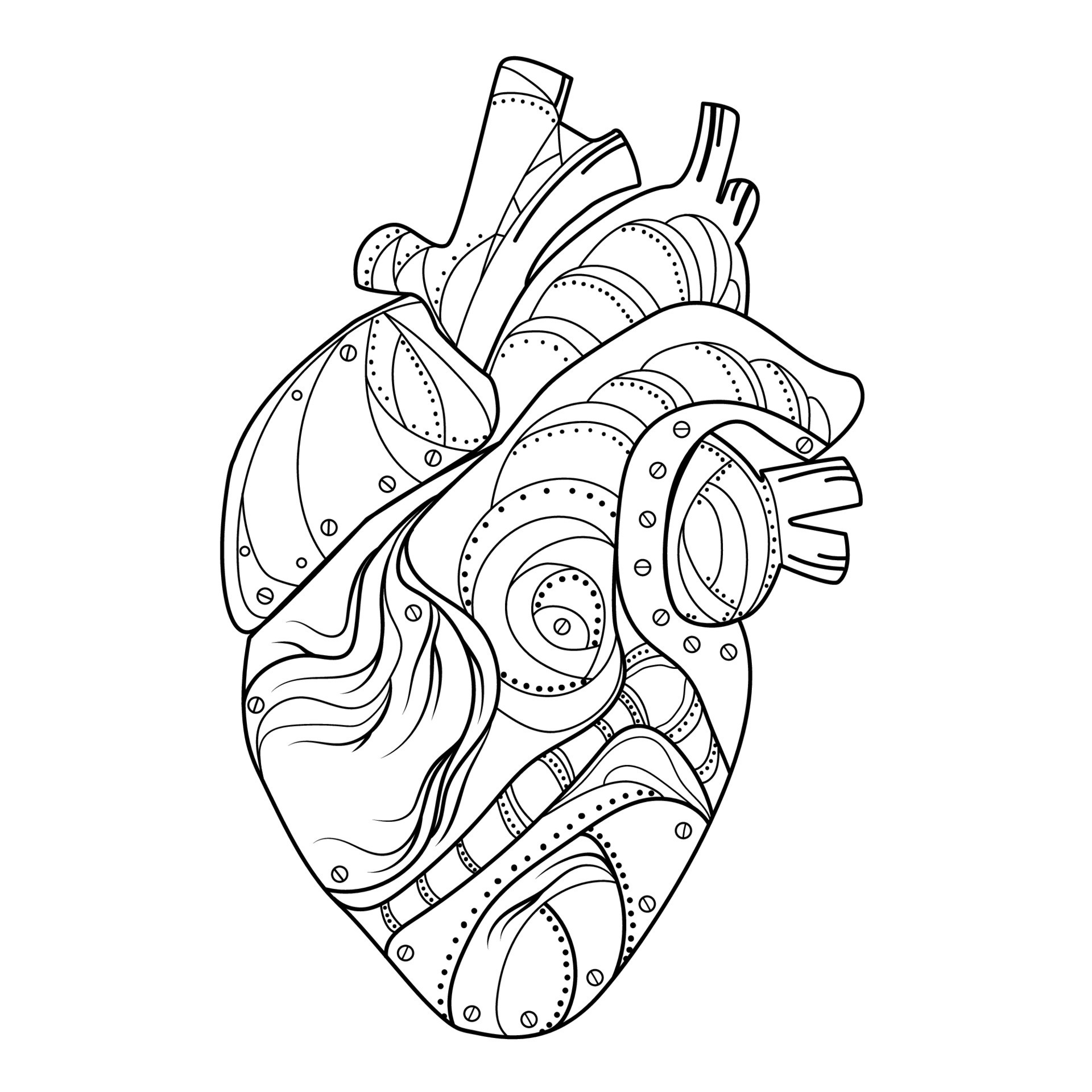A stylized black-and-white drawing depicts an anatomical heart, intricately detailed with various artistic elements. On the right side of the heart, multiple ventricles extend outward, adorned with sections featuring circular motifs, resembling rings adorned with small dots or rivets, sometimes appearing as tiny screws. Some portions of the heart are detailed with layered swirls, akin to folds of fabric, partially concealing the circular elements. Additionally, the ventricles and other parts extending from the heart are accentuated with parallel lines running along their outlines, adding to the complexity and depth of the illustration.